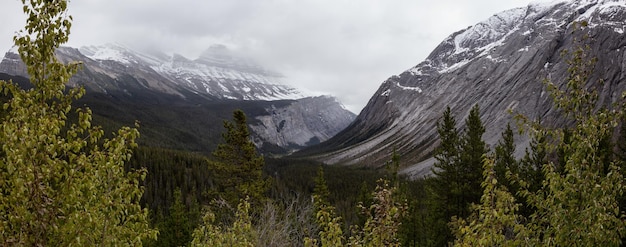This panoramic color photograph captures a breathtaking landscape of a forest and two towering, snow-capped mountains, likely glacially smoothed, rising majestically in the background. The mountain peaks, blanketed in snow, are shrouded by thick, white clouds that obscure the sky entirely, contributing to a hidden, almost ethereal atmosphere. Below the snowy crests, the dark gray mountain slopes extend down to meet a dense, vibrant forest comprised of both coniferous and deciduous trees that display varying shades of green. Some trees show signs of seasonal change or decay, hinting at the transition from fall to winter. The foreground is filled with these trees, including a notably dead bush, creating a rich tapestry of nature's cycles. Despite the weathered appearance of some foliage, the scene is unmarked by any signs of human presence or animal life, highlighting the untouched beauty of this serene wilderness.